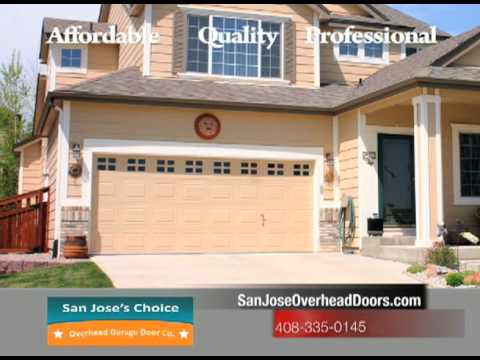A charming, spacious home with a single-door, two-car garage prominently features the message "Affordable, Quality, and Professional" in bold white lettering across the top. The house sports a unique tan exterior, which coordinates with the garage door color, creating an intriguing and cohesive aesthetic. Beneath the main slogan, the text "San Jose's Choice" appears in a vivid teal color, followed by "Overhead Garage Door Company" seamlessly integrated into the design with a sloping top. Adjacent to this, "SanJoseOverheadDoors.com" is displayed in dark charcoal lettering, clearly capitalized for readability. Below this, a contact number is set against a gradient of bright to pale pink. This inviting presentation conveys the reliability and excellence of the garage door company, encouraging visitors to trust them with their overhead door needs.